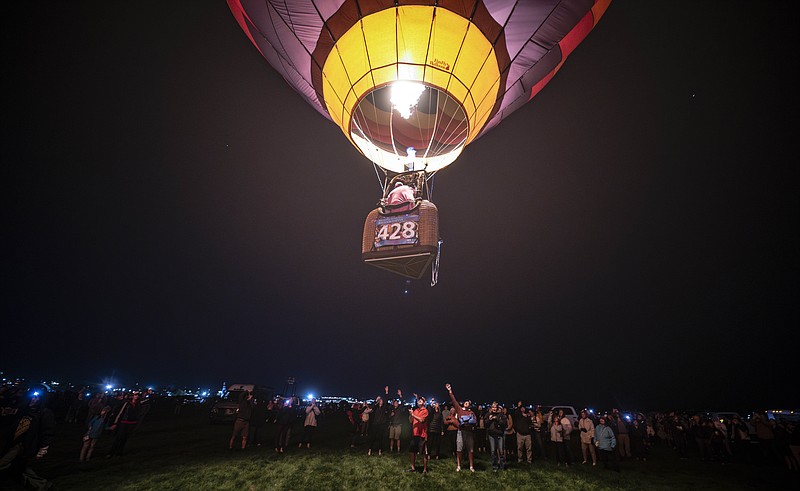In the photograph, taken at night, a vibrant hot air balloon ascends into the nearly black sky. The balloon, currently about 20 feet off the ground, is a kaleidoscope of colors with a bright yellow bottom bordered by shades of black, blue, red, burgundy, brown, and purple. Illuminated mostly by the intense flame within that keeps it aloft, the balloon's basket prominently displays the number "428." From this vantage, viewers can see the back of a person inside the basket. Below, a large crowd of people and cars, reminiscing a tailgate gathering, stands on a patch of green grass, gazing upwards. Many are gesturing excitedly at the balloon against a backdrop of distant lights from buildings along the horizon. The image captures the dynamic interplay of the balloon's vivid interior light and the deep darkness of the sky, highlighting a moment brimming with communal excitement.